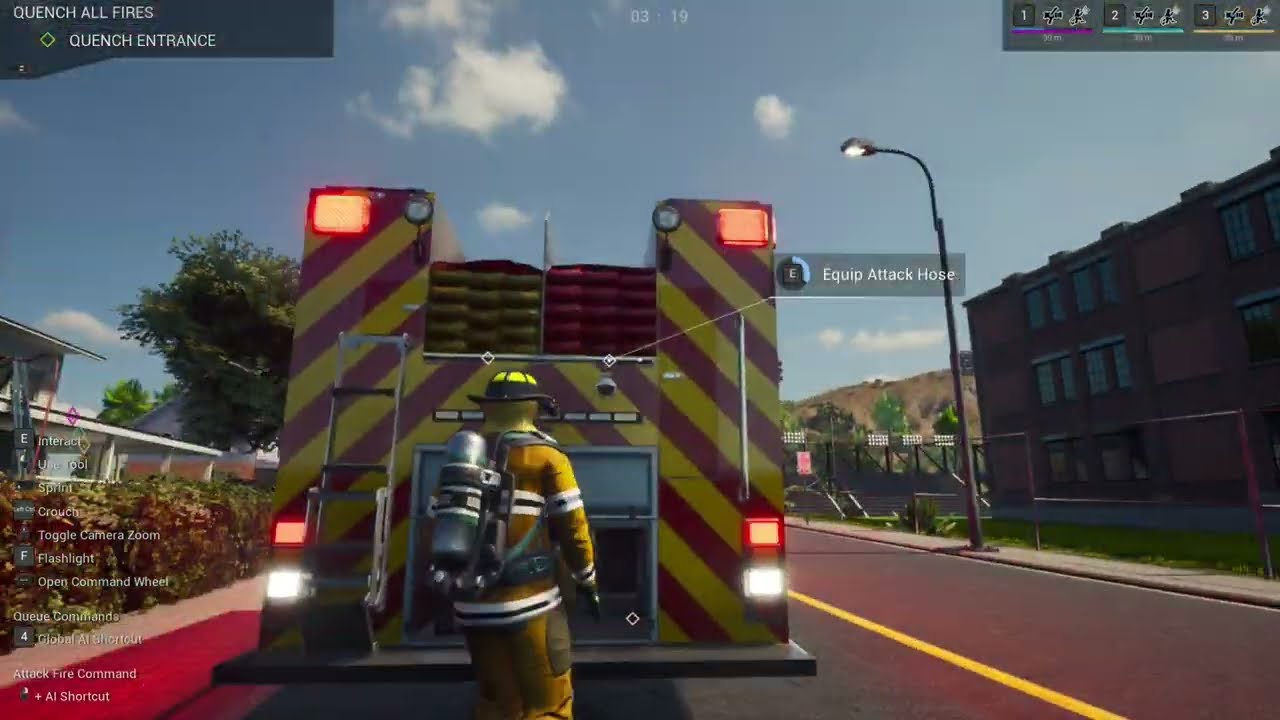In the image, captured from a third-person video game, a firefighter stands at the back of a fire engine adorned with yellow and red diagonal stripes. The firefighter, fully equipped in a tan uniform with high-visibility white stripes, wears a bright yellow helmet and has an oxygen tank strapped to their back. The fire engine itself features two prominent red lights at the top, along with taillights on the lower portion. Surrounding the scene, the street includes visible elements like a streetlight, buildings, and a yellow line on the pavement. In the distance, a hill suggests a Californian landscape under a hazy blue sky with a few clouds. Text boxes overlay the image, displaying messages such as "equipped attack hose" and "quench all fires, quench entrance" in the upper corners.